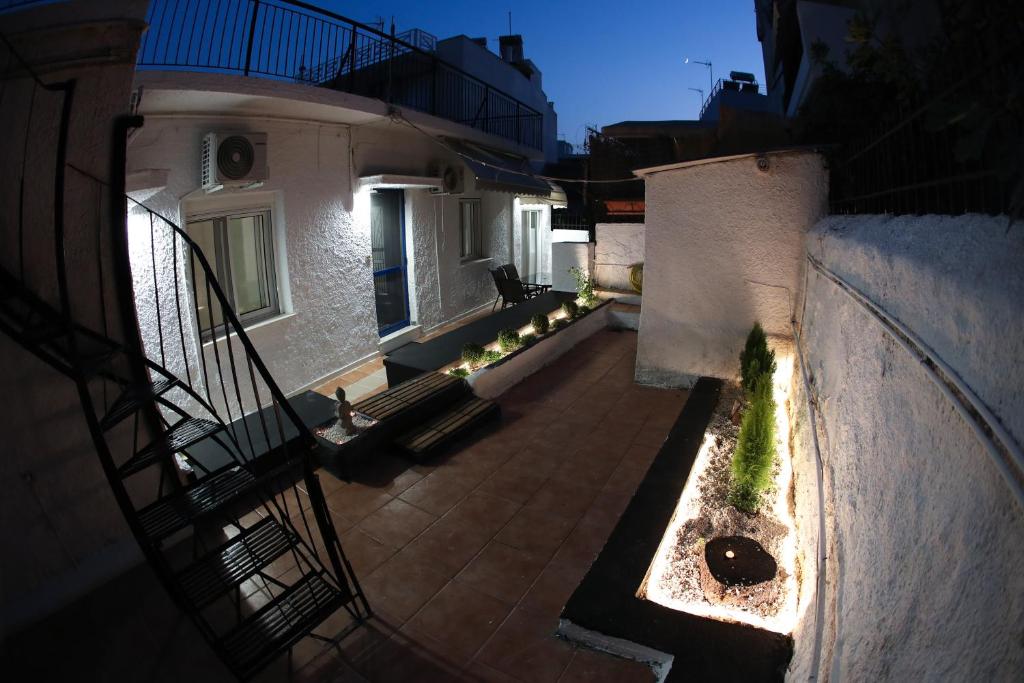This nighttime security camera image captures a peaceful courtyard scene, likely part of an apartment building or multi-level home. The courtyard features dark brown bricks and large brown paver stones across the ground. On the left side of the photo stands a spiral metal staircase ascending to a roof with a short railing. Adjacent to the staircase is a small patio area furnished with a couple of chairs. The right side of the image shows a planter with recessed lighting, illuminating both the plants and the brick wall behind it. Additional lighting can be seen in another small planter, enhancing the quiet, serene atmosphere of the area. There are no people present, contributing to the calm ambiance. In the backdrop, larger buildings can be faintly seen through the darkness, further contextualizing the courtyard within an urban setting.